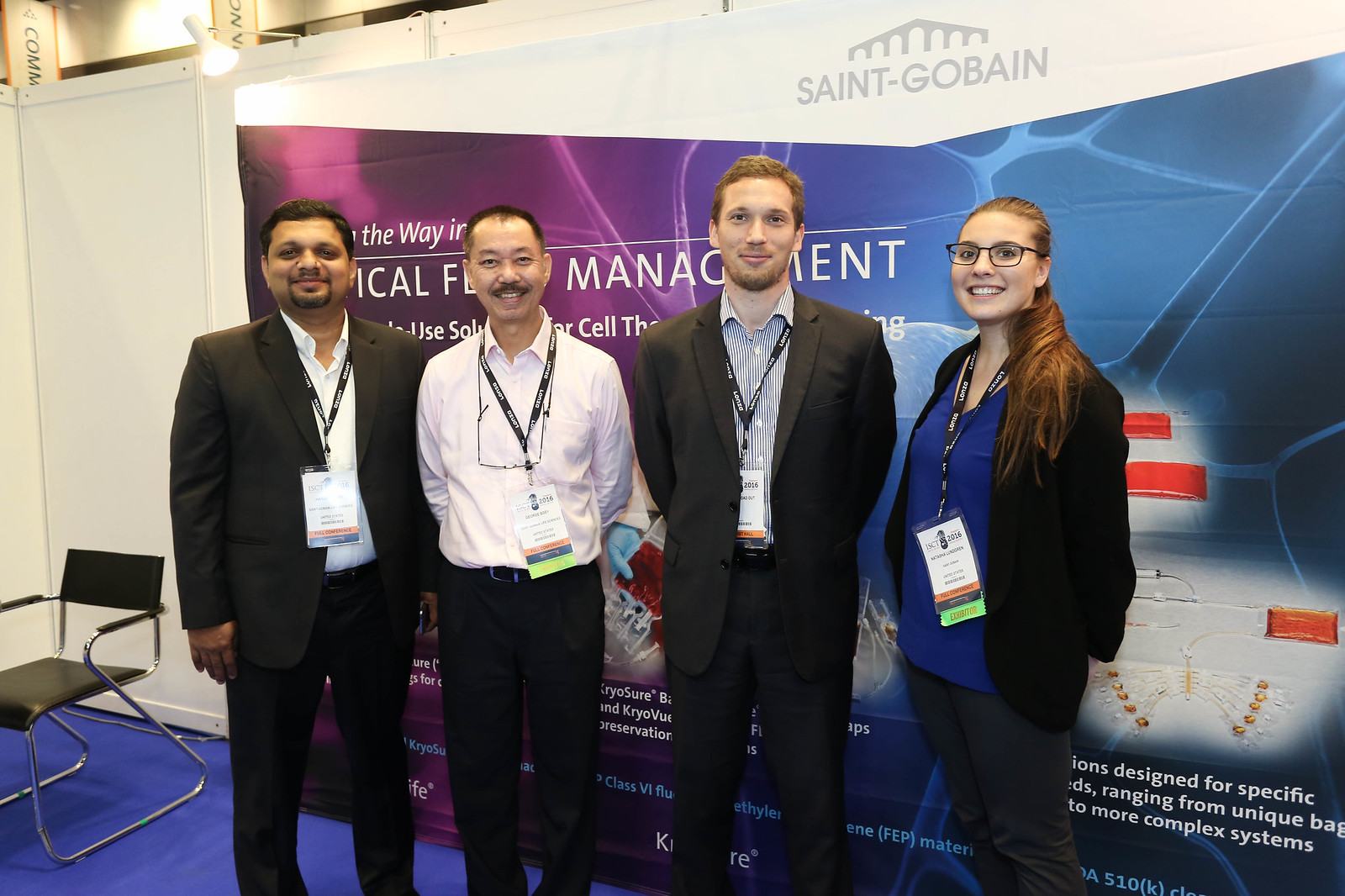The image is a full-color, indoor photograph taken at a professional event. It is rectangular in shape, wider than it is tall, and depicts four people standing in front of a backdrop. The backdrop transitions from purple on the left to blue on the right and features the partially obscured words "the way" and "management," with the logo "Saint-Gobain" prominently displayed at the top center in white and gray against a white background. The floor on the left side of the image is a purple-blue color, and a black chair is positioned in the far left corner. 

From left to right, the individuals are as follows:
1. A man with dark skin, short black hair, a black goatee, and a closed-mouth smile. He is dressed in a black suit over a white collared shirt and has a lanyard around his neck.
2. A man of Asian descent with lighter brown skin, wearing a white collared shirt, black pants, and also sporting a black mustache. He appears slightly older, is balding, and has a lanyard around his neck.
3. A younger, taller Caucasian man with light brown hair, a slight beard, and chin whiskers. He is dressed in a gray suit with an open jacket over a white and gray pinstriped shirt and also wears a lanyard.
4. A Caucasian woman with reddish-brown hair pulled back into a ponytail, black-rimmed glasses, and a bright smile. She is wearing a blue shirt under a black jacket and gray slacks, with a lanyard around her neck.

The scene is well-lit, highlighting the professional attire and demeanor of the individuals, who all appear to be engaged participants at the event.